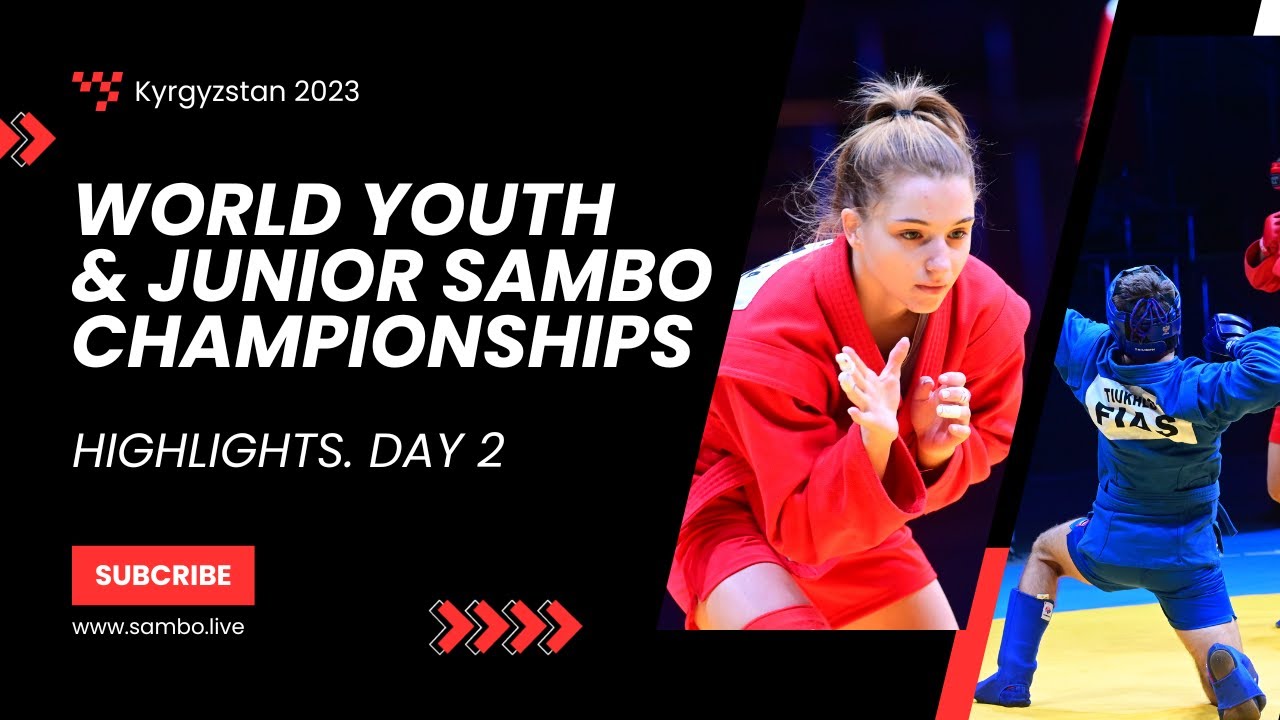The flyer is a rectangular, horizontally-aligned advertisement for the World Youth and Junior Sambo Championships 2023 in Kyrgyzstan. Set against a black background, the right side prominently features two athletes: a focused young woman with blonde hair in a ponytail, clad in a red martial arts uniform, standing in a fighting stance, and a young man viewed from behind, wearing a blue helmet, blue gloves, and a blue uniform with shorts, kneeling with one knee up. The left side of the flyer includes the event details— "Kyrgyzstan 2023" in white with a racetrack-themed red and black design beside it, followed by "World Youth and Junior Sambo Championships" in bold, all-caps white font. Below, in thinner white letters, it reads "highlights day two." The bottom left corner features a red "subscribe" button with "www.sambo.live" beneath it in small, white, lowercase letters. To the right of these details, four red arrowheads direct attention towards the images of the athletes.